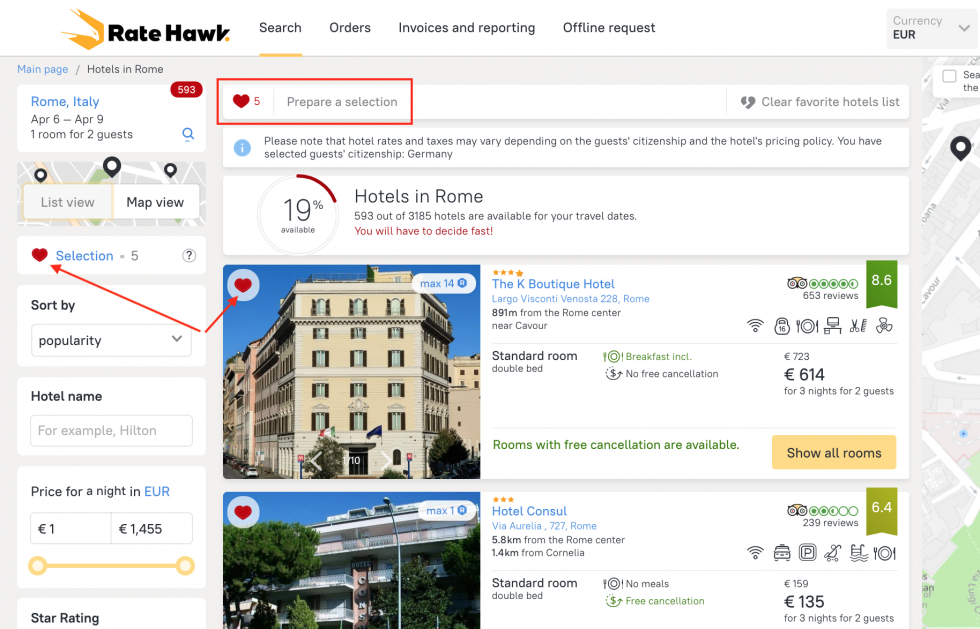This detailed caption provides an in-depth overview of the various options and details pertaining to a hotel booking for two guests in Rome, Italy, from April 6th to April 9th. It features information specific to the booking interface, such as categories like rates, hawk, search, orders, invoices, reporting, and offline requests. The currency is noted as euros. 

A notable point is that hotel rates and taxes may fluctuate based on the guest's citizenship and the hotel's pricing policy. For this booking, the guest citizenship selected is Germany. Out of 3185 potential hotel options in Rome, 593 hotels are available for these travel dates, comprising 19% of the total.

Two highlighted hotels include:

1. Cape Boutique Hotel, located in Lagobis County, Venezuela, at 228 Rome. It has a rating of 8.6 out of 10 based on 653 reviews.
2. Zekon Hotel Consul, located on Via Aurelia, 727 Rome. It has a rating of 6.4 out of 10 based on 239 reviews.